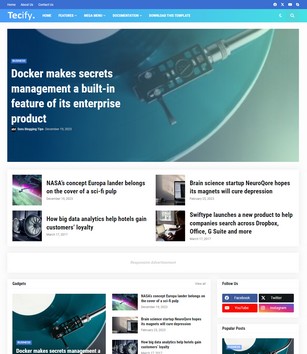This screenshot captures the mobile version of the TECIFY website. At the top of the page, the website's name "TECIFY." is prominently displayed. Below the title, an image of a vintage vinyl record player with a needle resting on a spinning record is featured. To the left of this evocative image, there is a headline that reads: "Docker makes secret management a built-in feature of its entire product." While the caption suggests some ambiguity about Docker and its offerings, the juxtaposition of the vinyl record might be more symbolic than literal, potentially highlighting the blend of old and new technology.

Further down the webpage, there are additional articles accompanied by thumbnail images. The text is small and somewhat challenging to read on this mobile layout. One article's headline discusses NASA's futuristic concept, suggesting an idea that belongs in the realm of sci-fi pulp fiction. Another nearby headline delves into how big data analytics are leveraged to enhance customer loyalty in the hotel industry. Overall, the TECIFY website appears to be a repository for diverse technology and science-related news and articles.